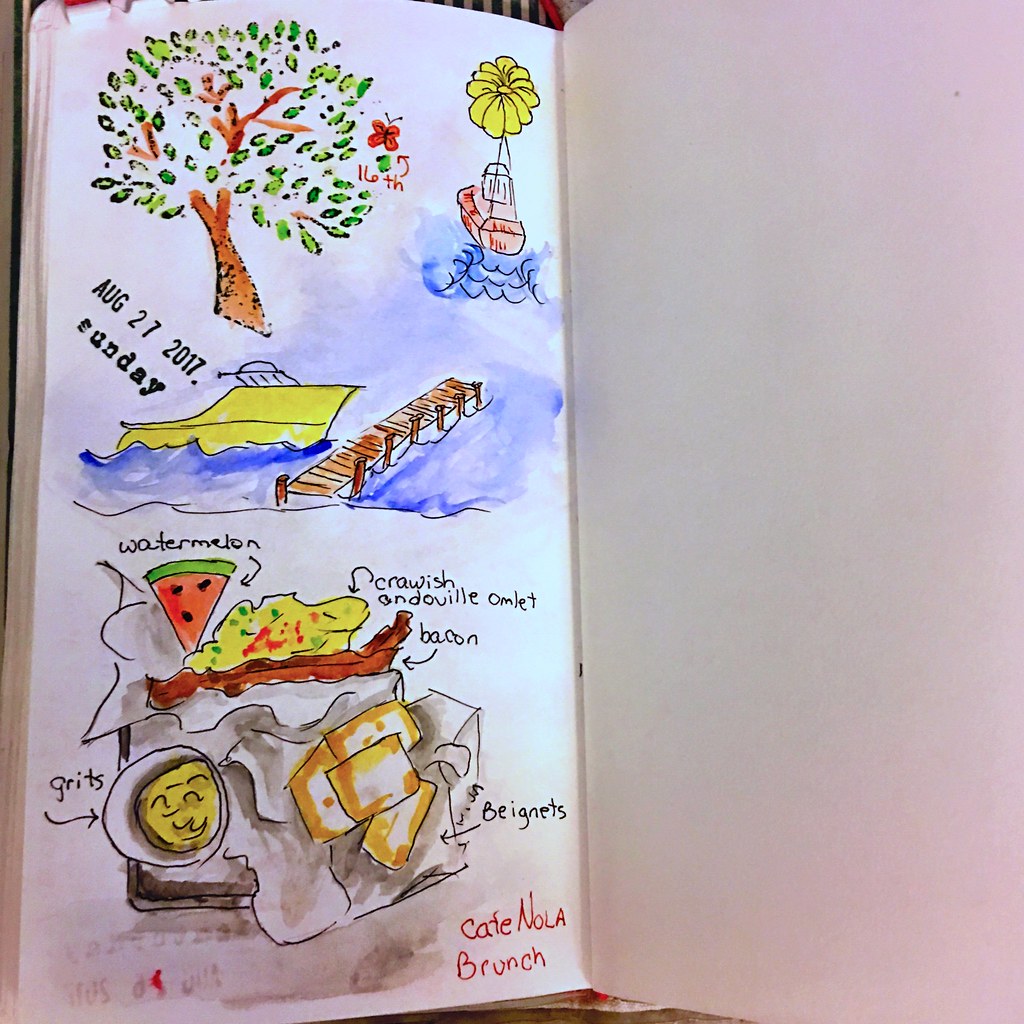A detailed photograph captures an open sketchbook diary featuring a collection of colorful drawings and handwritten notes chronicling a day's experiences. At the top of the page, the date "August 27th, 2017" is prominently displayed, marked in bold, stamped-like black letters with a hint of dark green. Adjacent to the date, a vibrant yellow boat sails on serene blue waters, accompanied by a textured brown wooden deck, symbolizing a Sunday boating adventure.

Beneath this nautical scene, the diary reveals a culinary journey from a visit to "Cafe Nola." The caption “Cafe Nola Brunch” indicates the setting for the meal, alongside intricately detailed illustrations of the dishes enjoyed. A juicy slice of watermelon, annotated with a black arrow and caption, is featured prominently. Below it, a crawfish and andouille omelet is depicted in rich colors, alongside crispy bacon strips, both meticulously labeled.

In the lower left section, a small bowl of golden-yellow grits sits in a pristine white container, while to the right, a stack of warm beignets dusted in a mix of orange, brown, and white hues takes center stage, each element carefully marked with arrows and descriptions in black ink. This diary page not only visually narrates a delightful day of exploration and dining but also showcases the artist's detailed and evocative style of documentation.